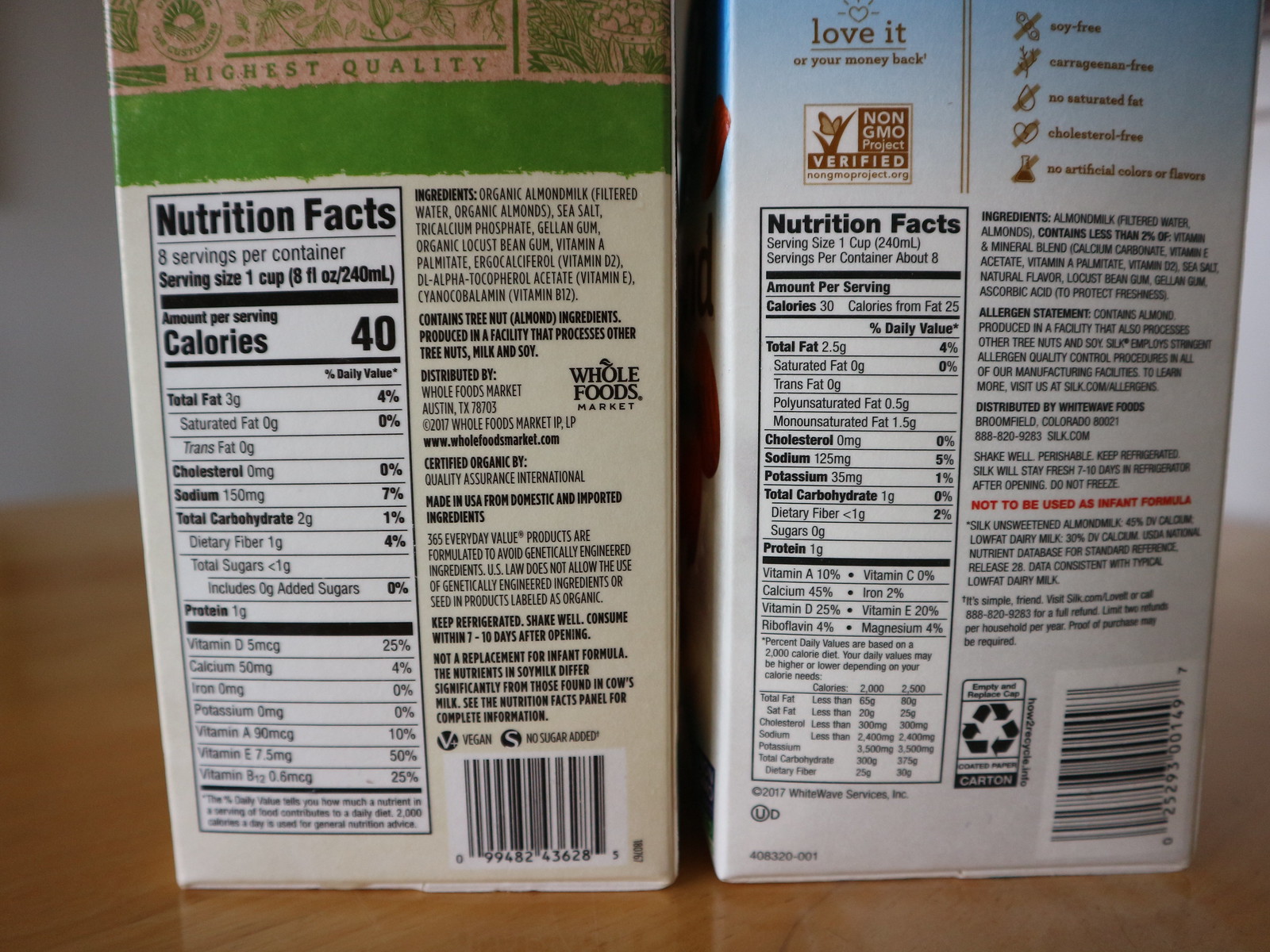The image shows the backs of two carton-like products that resemble milk cartons. Both cartons prominently display nutrition facts and ingredients lists. The carton on the left lists its primary ingredients as "organic almond milk," consisting of "filtered water" and "organic almonds," while the carton on the right simply states "almond milk," made from "filtered water" and "almonds."

The left carton features a brown top labeled with "Highest Quality" in a green strip. Its nutritional information notes that it contains 40 calories per one-cup serving. The right carton, with a blue top and brown text that includes the phrase "I love it or your money back," is marked as "Non-GMO Project Verified" and lists 30 calories per one-cup serving.

Both cartons have scanning labels located at the bottom right corner. They are positioned on a brown countertop against a plain white wall background, creating a clean and simple setting for the display.